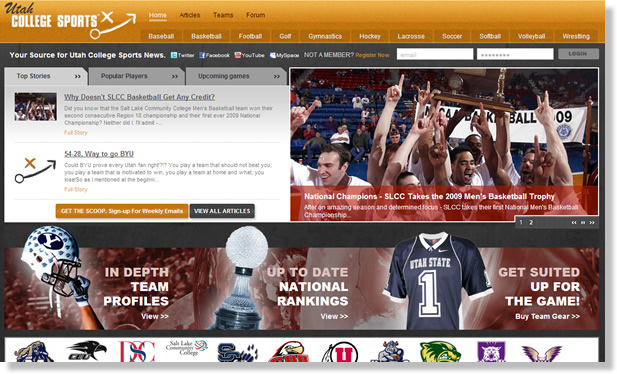**Detailed Description of Utah College Sports Homepage Screenshot**

The screenshot captures the homepage of the Utah College Sports website. Dominating the top of the page is a brown header. Positioned in the top left corner is the Utah College Sports logo. To the right of the logo are several navigation categories: Home, Articles, Teams, and Forum. Notably, the "Home" category is selected and highlighted with a white underline.

Directly beneath this header, a secondary navigation bar lists a comprehensive array of sports categories horizontally: Basketball, Baseball, Football, Golf, Gymnastics, Hockey, Lacrosse, Soccer, Softball, Volleyball, and Wrestling.

Below this navigation bar, a prominent black banner asserts, "Your source for Utah coverage begins here." This banner includes hyperlinks to social media accounts: Twitter, Facebook, YouTube, and an additional unspecified platform.

On the right side of the page, adjacent to the banner, are two text boxes for user name and password entry, accompanied by a button to log in.

The main body of the website is filled with various articles detailing different sports teams, providing extensive coverage on Utah college sports.